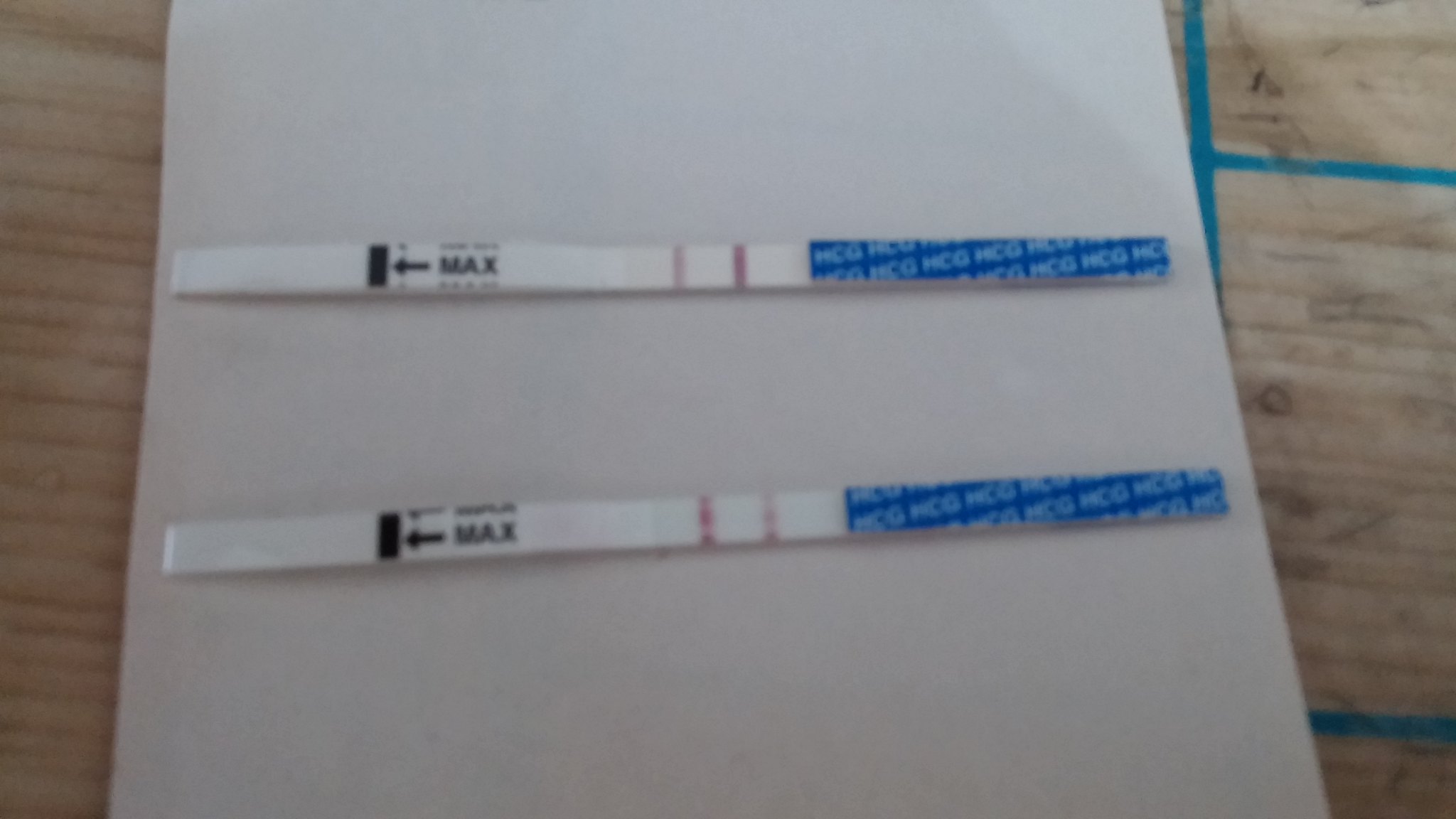The image depicts two pregnancy test strips laid out on a piece of white paper, placed on a wooden table adorned with faint blue lines. These test strips, commonly purchased from a pharmacy, work by detecting the hormone Human Chorionic Gonadotropin (HCG) in a woman's urine—a key indicator of pregnancy. When a woman urinates on these strips, the presence of elevated HCG levels causes a color change, typically manifesting as an additional line to signify a positive result. The right side of each strip features white lettering on a blue background that reads "HCG," denoting the specific hormone tested. This hormone's concentration increases as pregnancy progresses, making these strips a reliable method for indicating early pregnancy.